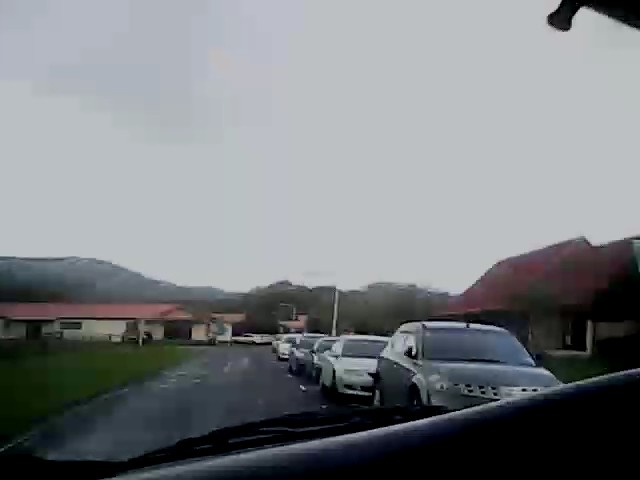A photograph taken from the passenger side of a car in Europe shows a vivid scene through the windshield. The wiper blade and edge of the dashboard are visible, indicating the car's interior perspective. The vehicle is driving on the left side of the road, with a line of oncoming traffic to the right. Leading the traffic is a bluish SUV, followed by four or five smaller cars stretching into the distance. The road is paved with gray asphalt, marked by a white dotted line in the center.

On the left side of the road, overgrown wild grass borders the gray expanse. In the middle distance, a tan building with a reddish roof stands, with several cars parked in front of it. The scene extends to a backdrop of a hazy mountain range and patches of green trees under an overcast, light blue sky. To the right, another building with a pointed red roof adds to the architectural elements. The entire image has a slight blur, contributing to a hazy atmosphere.